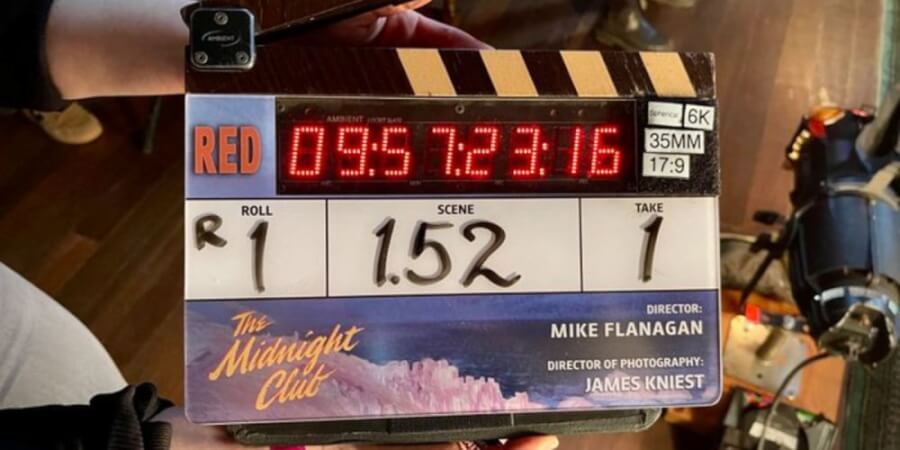In this detailed image, we see a man holding a traditional film clapperboard, commonly used to mark scenes during filming. The top of the clapperboard features a black section with diagonal yellow stripes. On this black section, there's a blue background square with the word "RED" in red font. Just below, a digital display shows the timestamp "09:57:23:16", flanked by "6K, 35mm, 17:9" to the right. The main body of the clapperboard has the details: "Roll R1, Scene 1.52, Take 1," and below that, in yellow cursive on the left, it reads "The Midnight Club," with the credits "Director: Mike Flanagan" and "Director of Photography: James Knist" in white on the right side. Off to the right side of the image, a staging light can be seen, indicating that a scene is about to be filmed.